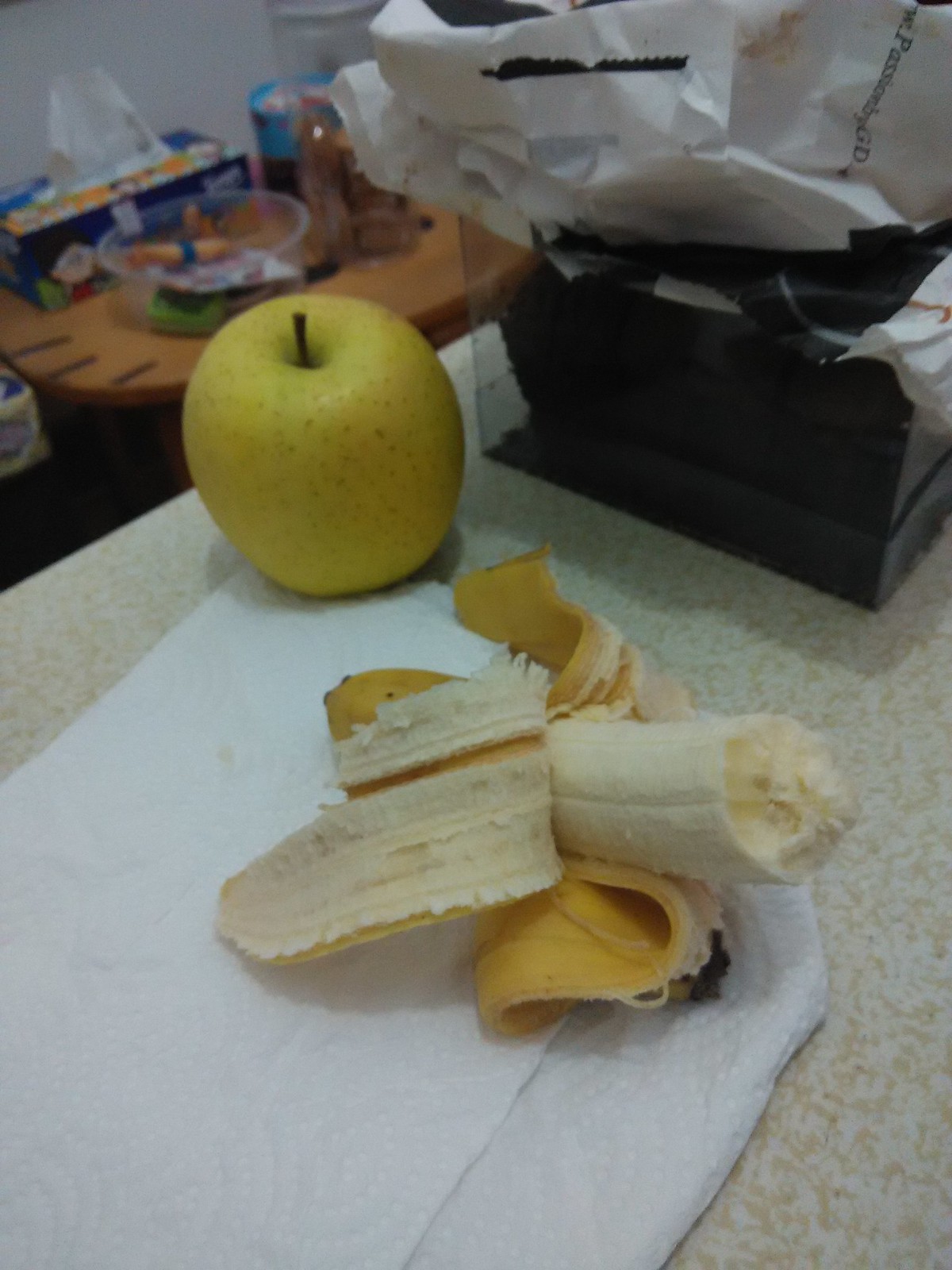In the image, a white countertop with subtle yellow marbling serves as the backdrop. Resting on the countertop is a white paper towel, occupying a central position. On the paper towel lies a half-peeled, half-eaten banana. Adjacent to the banana, at the corner of the paper towel, is a whole green apple with its stem still attached.

Above these fruits, a clear container filled with an indiscernible black substance is visible. On top of this clear container, several paper bags or packages are stacked, possibly containing food items.

In the slightly blurred background on the top left, a small wooden table, likely oak, can be seen. On the table sits a box of tissues alongside several clear containers that hold an assortment of unspecified items, with one resembling a pretzel bin. Additionally, on the left side of the oak table, three black lines run vertically, which appear to be strips of tape or similar material.